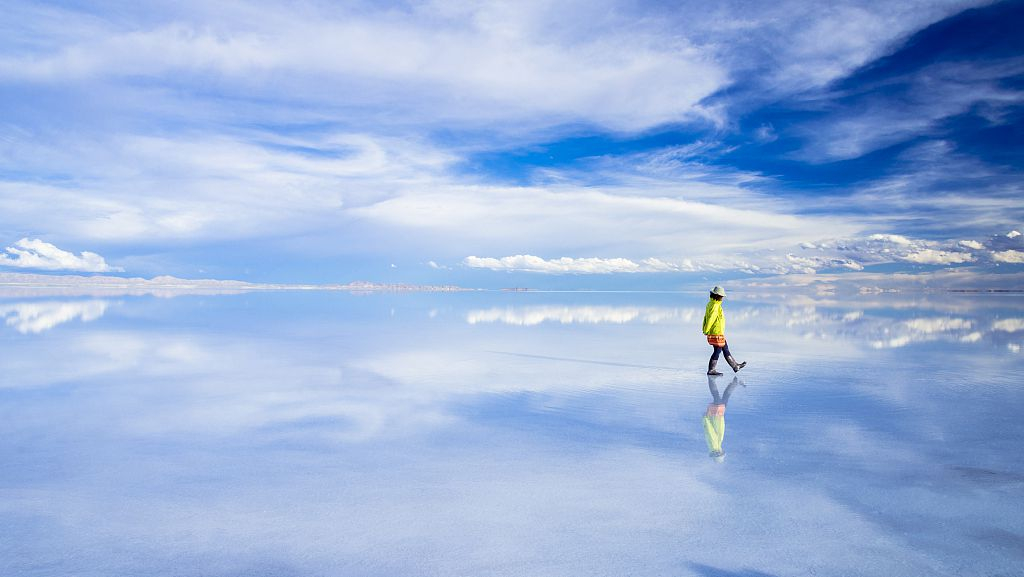In this surreal photograph, a dramatic and ethereal outdoor scene is captured, where the ground perfectly mirrors the sky, creating an illusion of walking on the sky. The setting appears to be a vast expanse of shallow water stretching out to the horizon, where the water's surface reflects the dark blue sky streaked with thin white clouds, making the ground indistinguishable from the sky. In the foreground, a person clad in a bright yellow raincoat, white hat, and black boots is either walking or kicking at the surface, seemingly floating in this dreamlike landscape. The individual’s reflection on the water enhances the illusion of walking on the sky. Towards the center of the image, a thin line of light gray rocks runs from the left and down the center, adding a touch of symmetry to the scene. In the far distance, hints of mountainous land can be seen faintly on the left and right sides of the horizon, blending seamlessly into the endless sea of water and sky.